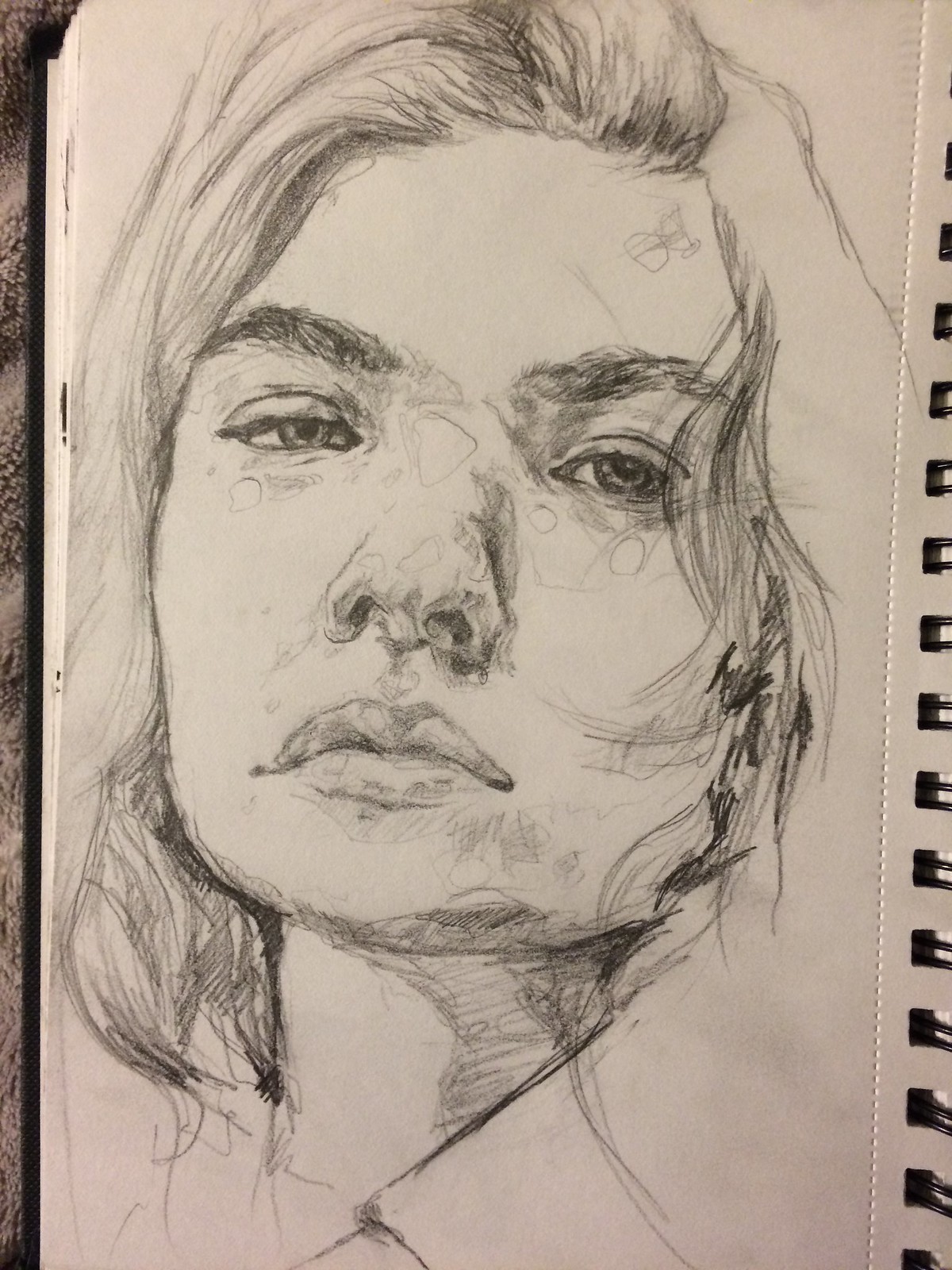This black-and-white image features a detailed drawing of a woman's face, centrally positioned on a piece of white paper. The woman's facial expression is calm, with her eyes looking straight ahead. The finely rendered hair frames her face and extends down to her neck. On the right side of the image, the spiral binding of the sketchbook is visible, indicating that the drawing is part of a bound collection. Additionally, a faint cutting line is noticeable to the left of the spiral. The intricate details of her nose, lips, and hair strands highlight the artist's meticulous work.